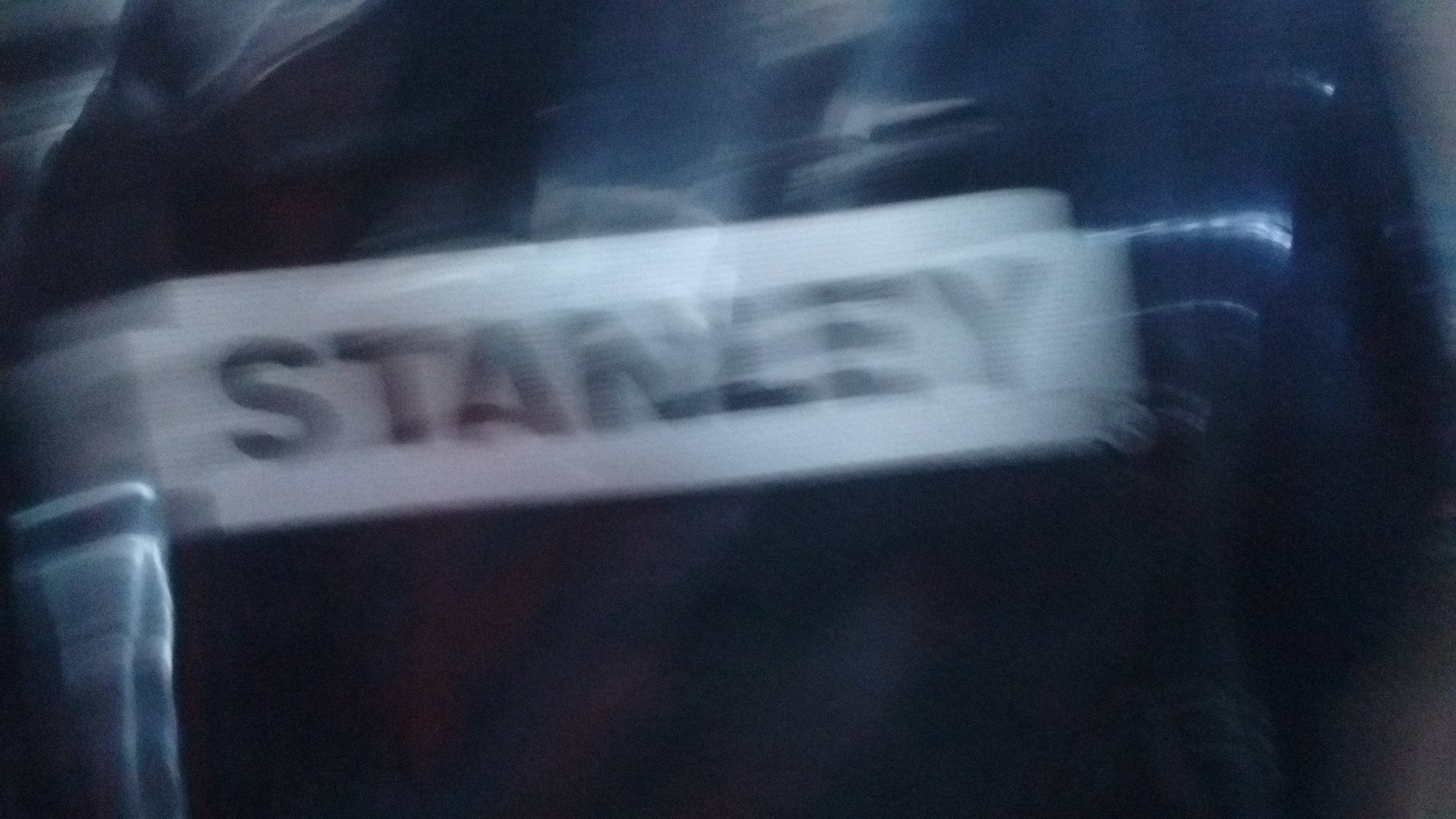A blurred photograph featuring a close-up view of a label on what appears to be a dark piece of clothing. The motion blur makes the white rectangular label difficult to read, but it seems to have the word "Stanley" printed in black text. The fabric of the garment appears to be a dark blue, possibly black, with hints of white stripes faintly visible in the image.